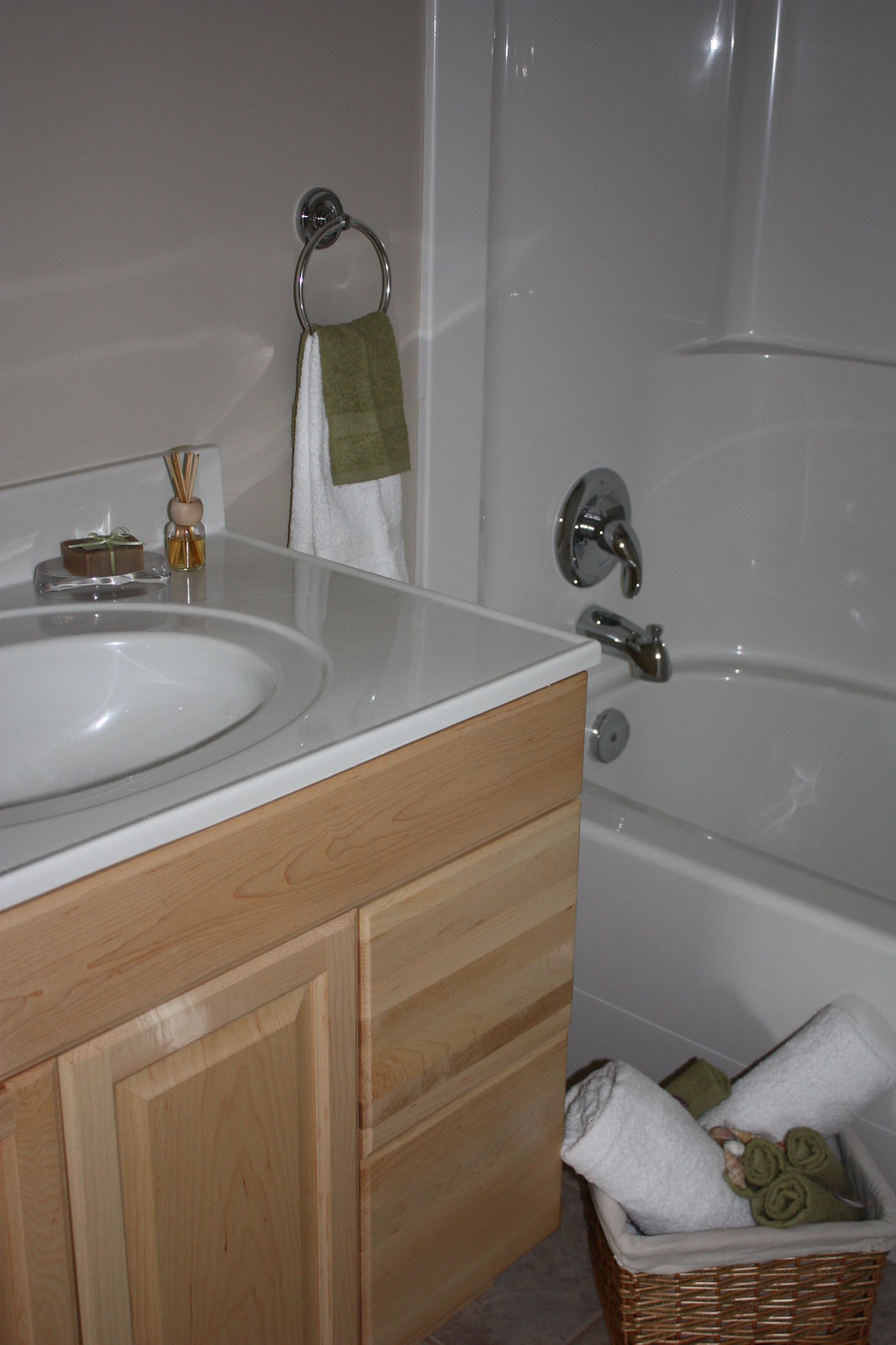The photograph captures an impeccably clean and neatly organized bathroom. On the left side of the image, there is a pristine white bathtub, gleaming under the light with shiny handles and knobs. The shower curtain appears to be pulled back, rendering the full bathtub partially out of view. Adjacent to the tub, a silver round towel rack holds a pristine white towel accompanied by a smaller green hand towel. 

In the bottom left corner, a charming wicker basket with a white fabric insert contains two thick white towels and four neatly folded green hand towels. The sink area features a spotless white basin set into a light brown wooden cabinet with two drawers and a cupboard beneath. On the sink counter, a soap dish and a small bottle with fragrance sticks add a touch of elegance to the space. The bathroom, although compact, is immaculate and exudes a sense of tranquility and cleanliness.